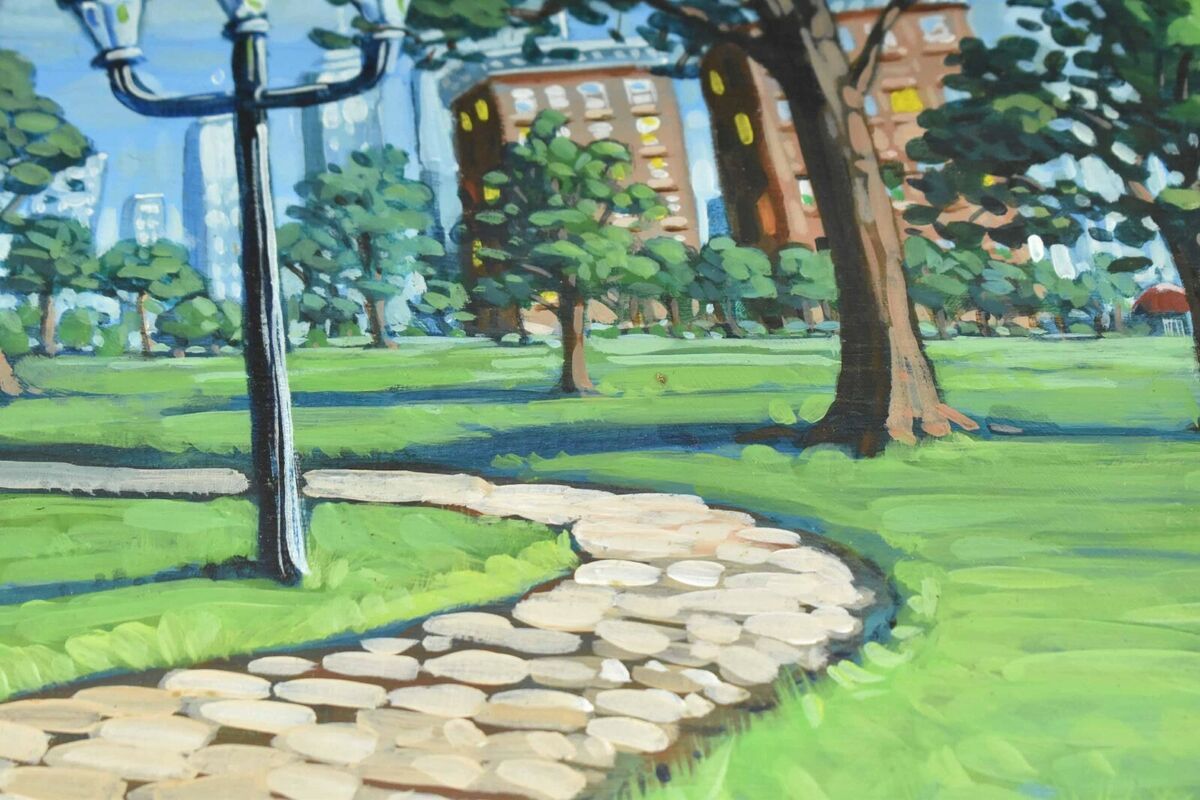This animated painting vividly captures a serene daytime scene in an urban park. The foreground is dominated by a curving cobblestone walkway that occupies the bottom left and winds around a distinctive lamppost. This black and silver streetlight features three lanterns—one at the top center and two extending from side arms. The path is bordered by lush green grass, which spreads across the scene. On the right side, a large tree with a sturdy brown trunk stands among several smaller trees, all thriving with green leaves. The backdrop includes an assortment of buildings. Prominently, there are two tall white office buildings and adjacent to them, a larger, wide brown structure accented with white and yellow hues. Further left, the city skyline emerges with towering skyscrapers that glisten in silver tones. This park, presumably a city park, offers a charming blend of natural beauty and urban architecture, set against the backdrop of an inviting sky.